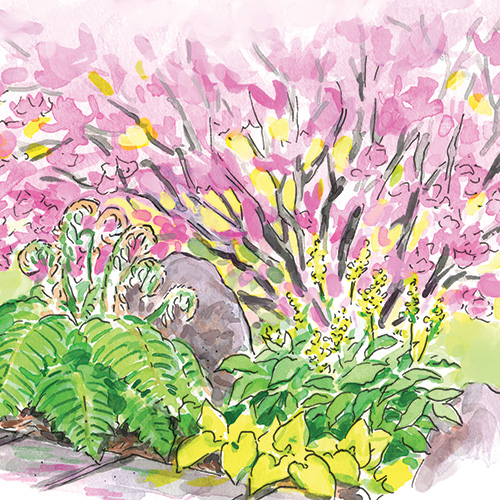This artwork, possibly a watercolor painting, is set within a square frame and depicts a lush, vibrant garden scene. The foreground features a combination of intricate ground covers—yellowish blooms or leaves and green, fern-like plants, with prominent spore-bearing fronds on the left. The base of the scene is anchored by a paved stone pathway composed of square segments, primarily white with subtle pink and green highlights. This pathway occupies the bottom left corner of the frame. Dominating the middle ground, a large gray boulder is nestled among the vegetation. Flanking this central element, hostas and other greenery support tall spikes of yellow flowers. In the background, a large bush or tree spreads its branches, laden with pink and yellow flowers that blanket the upper part of the composition, enhancing the overall lushness of the garden. The piece is rendered with a mix of loose, abstract strokes and partial black outlines, contributing to its dynamic and expressive nature.